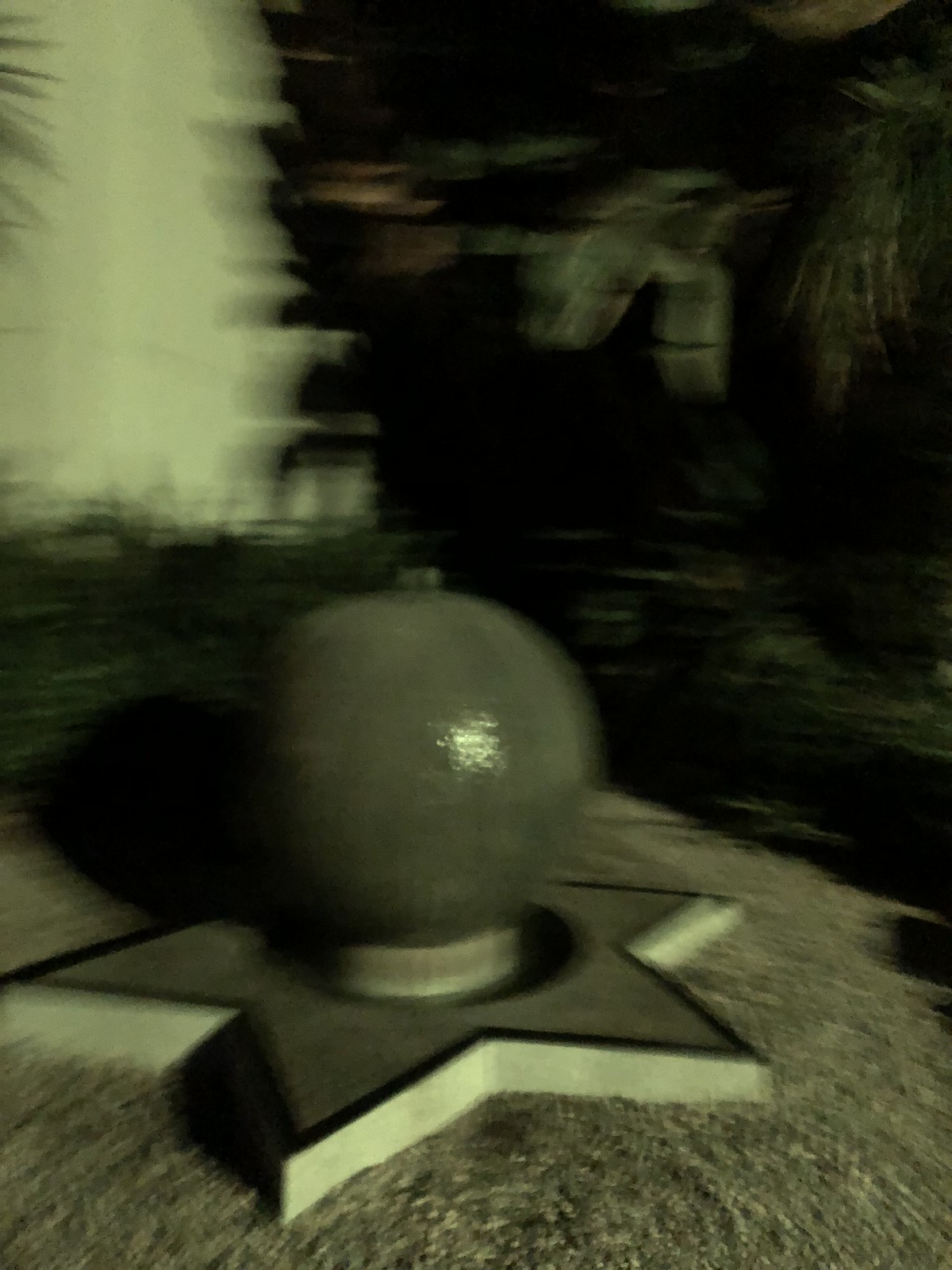This blurry daytime photograph captures a water fountain with an unusual star-shaped cement base surrounded by gravel. In the center of the star, a large, wet sphere emerges, with water visibly cascading down its surface and collecting in a small receptacle at the bottom. Despite the overall blurriness, low bushes can be seen around the fountain. The lighting and shadows create a peculiar visual effect, with dark splotchy bits and shadows cast on the nearby wall, contributing to the indistinct and somewhat surreal ambiance of the scene.